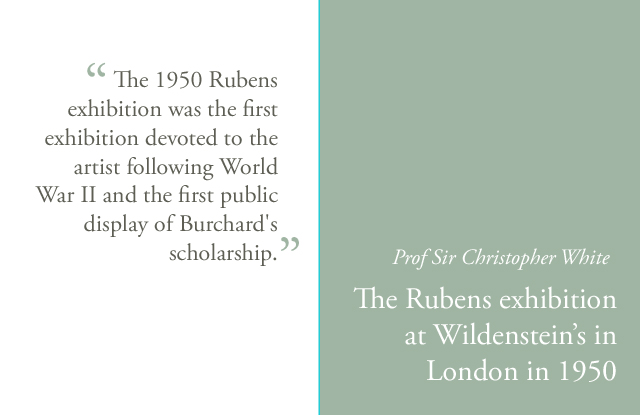The image is of an informational digital slide split into two equal halves. The left half is a white rectangle bordered by a very thin, light blue line in the center, and the right half is a green rectangle. On the left side, enclosed in green parentheses, black text reads: "The 1950 Rubens exhibition was the first exhibition devoted to the artist following World War II and the first public display of Burchard's scholarship." On the right side, towards the bottom of the green rectangle, white italicized text reads: "Professor Sir Christopher White. The Rubens exhibition at Wildenstein's in London in 1950." The entire slide features a cohesive color scheme of green and white, with a subtle light blue divider accentuating the separation between the two segments.